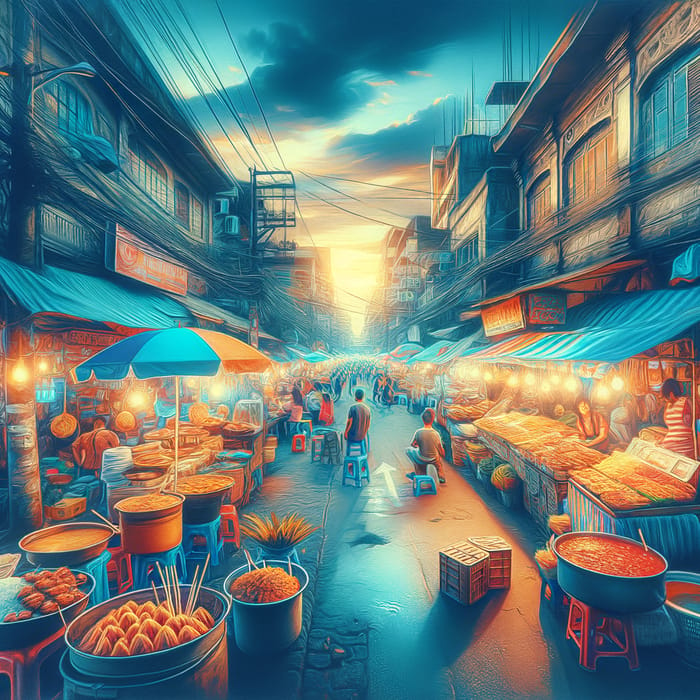This painting is a vibrant, hyper-realistic depiction of a bustling marketplace, likely set in a historical or underdetermined timeframe, reminiscent of scenes you might find in places like India. The setting is a narrow street or alleyway, flanked by two-to-four-story buildings. The artist uses a striking palette dominated by shades of orange and blue, imbued with an orangey-green glow, suggesting a sunset scene with light filtering through scattered clouds. The street is teeming with activity: vendors with booths and market stands line both sides, sheltered by awnings and colorful umbrellas. There are numerous pots brimming with vivid red and orange foods, including chili, chicken, and fish. Crates and chairs are scattered around, with people of all ages either sitting or walking, absorbing the lively atmosphere. Electrical wires crisscross overhead, adding to the dense, layered feel of the marketplace. The painting captures the essence of a busy, vibrant community hub bathed in the warm hues of twilight.